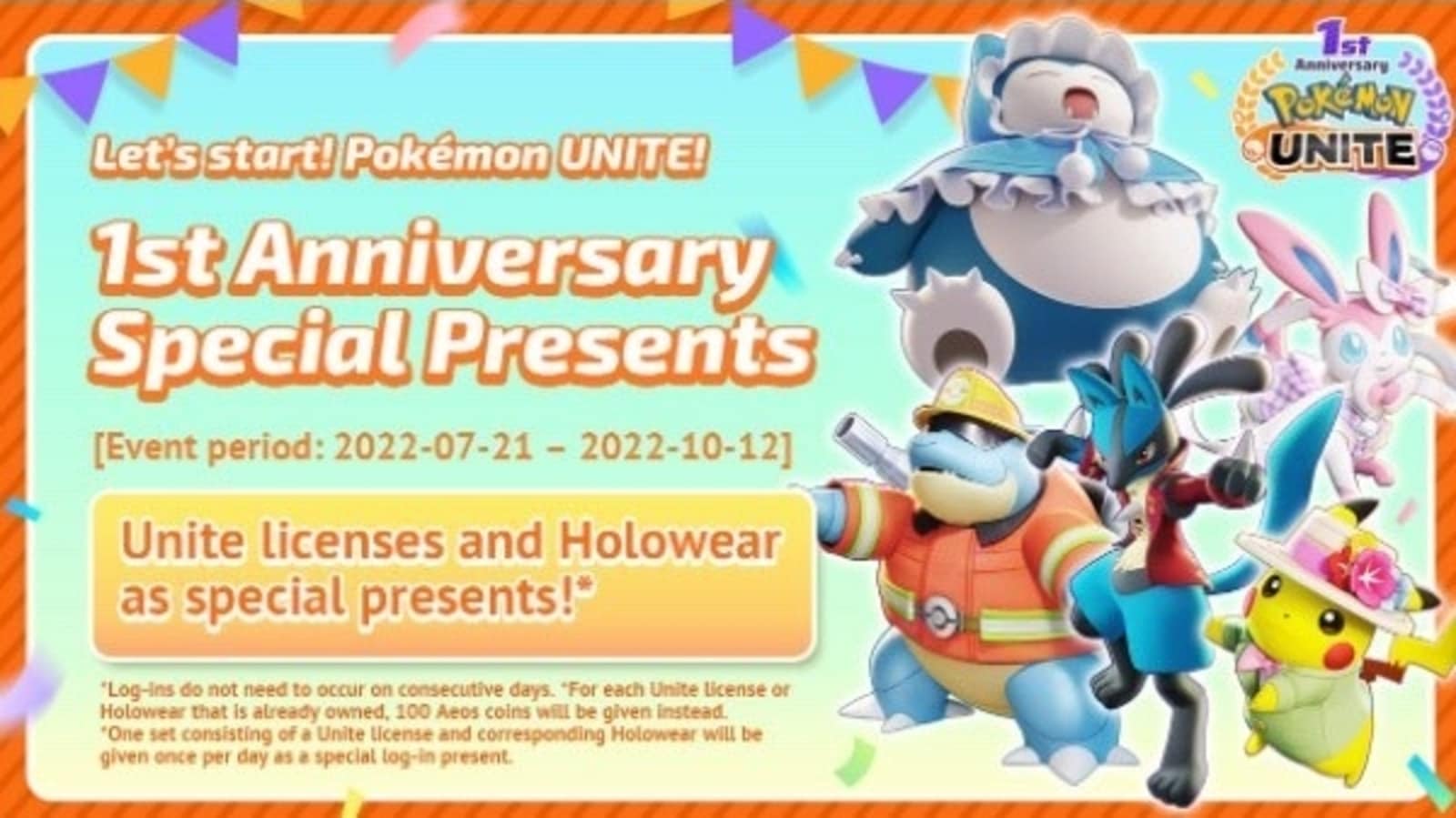"Commemorating the first anniversary of Pokémon Unite, this dynamic poster invites players to celebrate with special presents, including Unite Licenses and Holowear. The event runs from July 22 to October 22. Prominent Pokémon, detailed in three-dimensional graphics, grace the right side of the poster. Recognizable characters such as Pikachu, Blastoise, and Snorlax are featured alongside newer generation Pokémon. Each Pokémon is adorned in customizable outfits, highlighting Pikachu in a charming pink bonnet decorated with flowers and Blastoise in a fireman’s helmet and torso gear. The bottom of the poster includes legal details pertinent to the event."